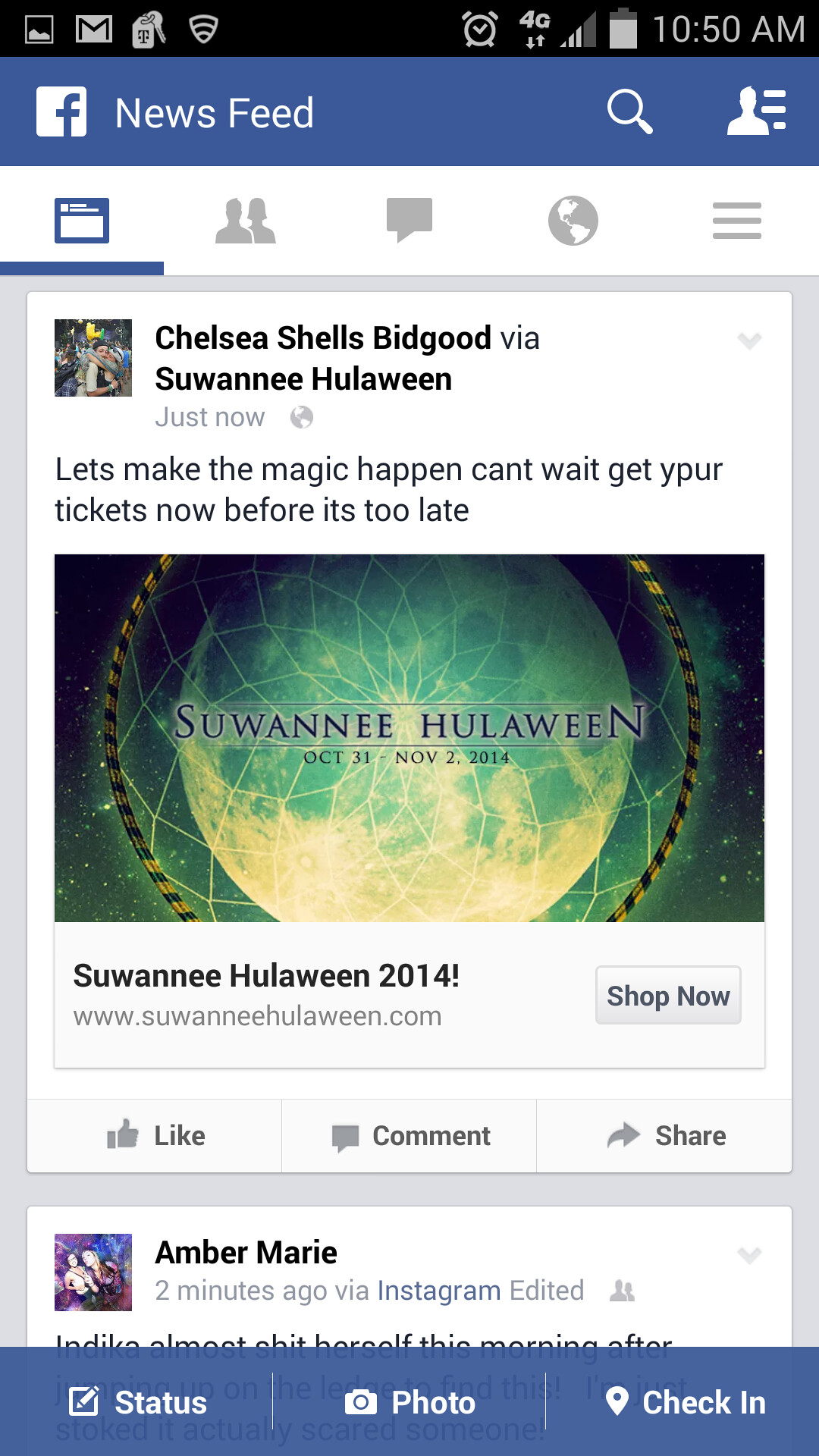This screenshot shows the Facebook News Feed on a mobile phone at 10:50 AM. At the top, various status icons indicate T-Mobile reception, 4G signal, battery level, and notification symbols. Below the Facebook logo and "News Feed" header, the main content features a post by Chelsea Schell’s Bread Good via Suwannee Hulaween, made just moments ago. The post enthusiastically announces, "Let's make the magic happen, can't wait, get your tickets now before it's too late," accompanied by an event notice for "Suwannee Hulaween 2014," which runs from October 31st to November 2nd, 2014. The event notice showcases an image of a geometric, glowing green globe. Below this post are interactive buttons for like, comment, and share. A subsequent post by Amber Marie, shared two minutes ago via Instagram and noted as edited, partially appears below. The bottom of the screen displays options to update your status, add a photo, or check-in, set against a blue background.